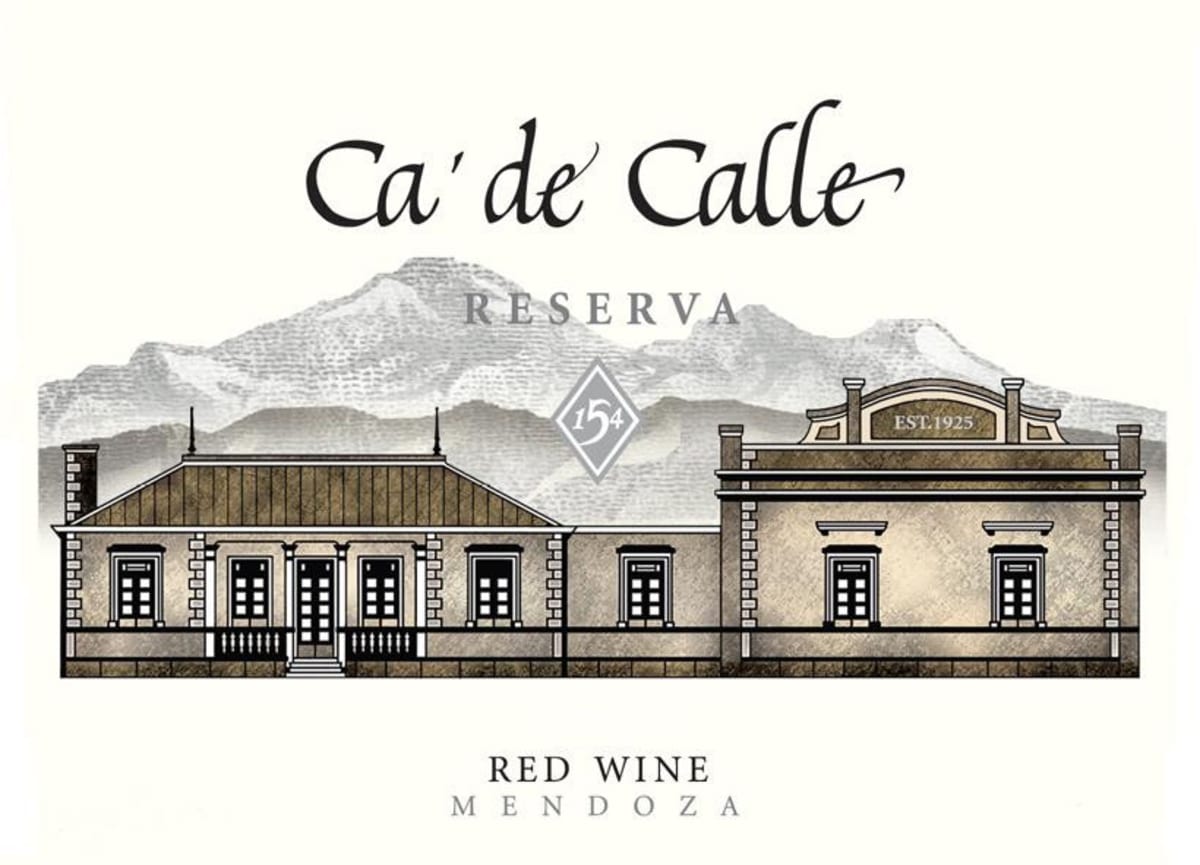The image features a detailed, hand-drawn wine bottle label with a predominantly pen illustration against a pale cream background. The central focus is the name "Catecalle," elegantly scripted in a scrawled font. Beneath this, the word "RESERVA" is prominently displayed in grey capital letters with a subtle mountain range backdrop. The center of the label showcases a diamond motif in white and grey, emblazoned with the number "154." Below these elements is an intricate illustration of a historic building, characterized by its detailed brickwork, plasterwork, unique chimneys, and turrets. The building has multiple windows, a small set of steps leading to the entrance, and a walled-off area at the front. Notably, the right side of the structure features an inscription reading "Established 1925." The label concludes with the designation "Red Wine, Mendoza," presumably indicating the wine's origin or specialty.